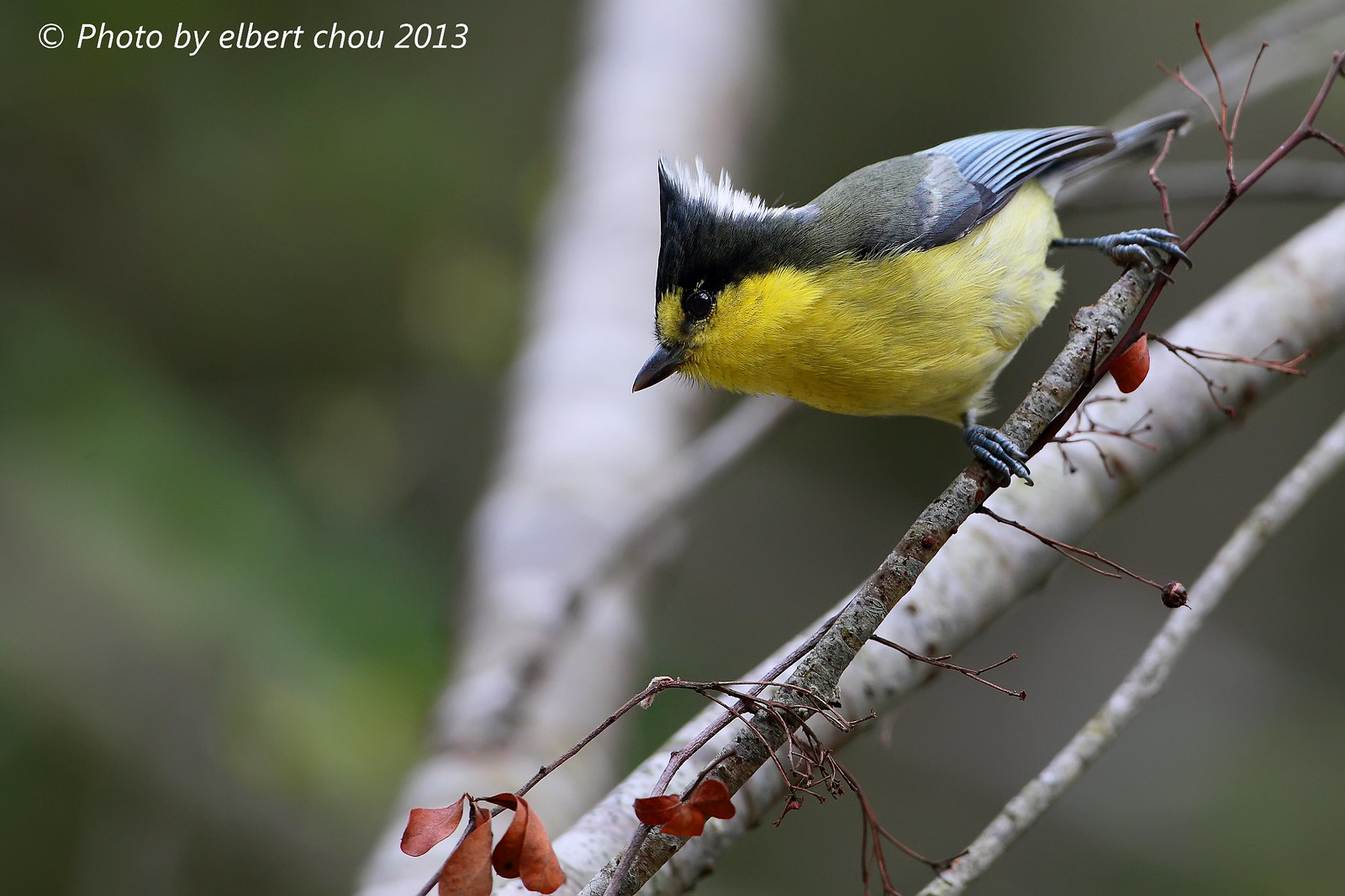This detailed close-up image showcases a striking bird, predominantly yellow with brownish and white accents. The bird's head features a distinctive pointed crest of feathers, giving it a mohawk-like appearance, with the white feathers adorning the back of its head. The bird has a prominent, large eye, and a small brown beak. It clings to a dead, brown branch with its little gray legs. 

The bird's lower half is gold, while the top half, including its head and wings, displays shades of darker, black feathers. The background of the image is intentionally blurred, accentuating the bird while creating a soft focus effect. It reveals a mix of green hues, potentially from grass or trees, and gray areas. Additionally, white branches are visible, some with red berries or leaves hanging from them, creating a contrast against the otherwise neutral backdrop.

In the top left corner, the image bears a copyright notice in small, white print, reading: "Copyright photo by Albert Chow 2013."